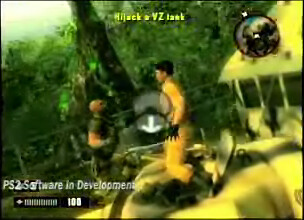This image appears to be a still from a video game. At the top of the screen, the text "Hijack a VZ Task" is displayed, albeit slightly out of focus. Along the bottom, the words "PS2 Software and Development" are visible, accompanied by a life bar that reads 100. The scene is set in a jungle environment, featuring two characters standing in front of a fence and atop a vehicle. 

To the right of the scene, there's a building, with lush greenery and a tree visible in the background, extending up to meet the sky. One character, dressed in yellow, is seen stepping out of the vehicle. At the center of the screen, a white downward-pointing arrow is present. To the left of this arrow stands another character, who appears to be bald and clad in green combat fatigues. The detailed setting and characters evoke a vivid, action-packed atmosphere typical of PlayStation 2 video games.